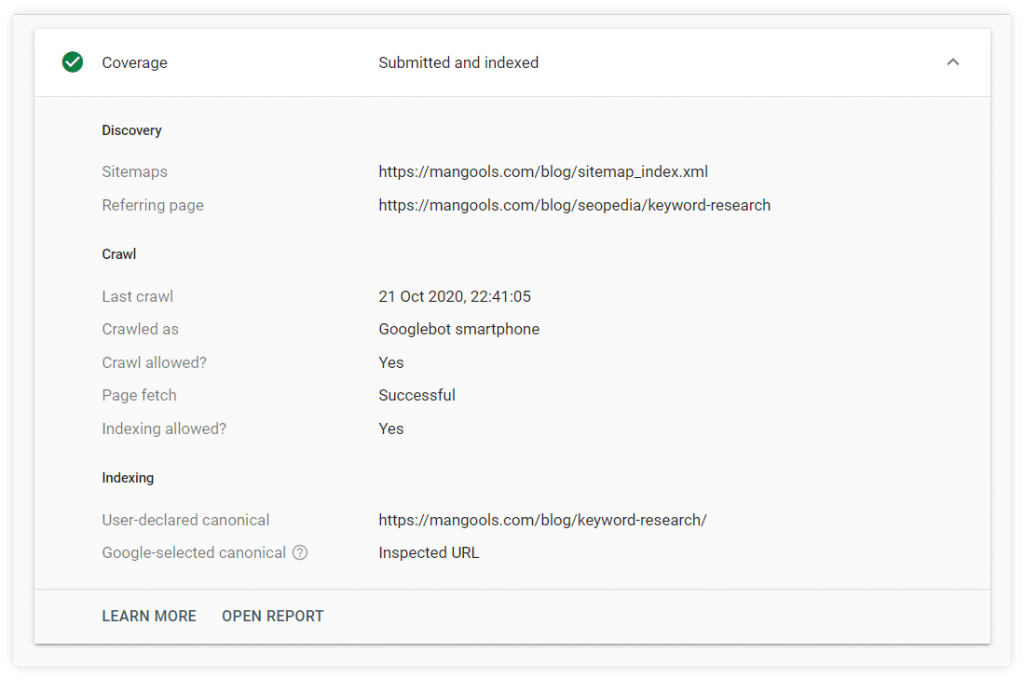This screenshot appears to be from a website analysis tool, showcasing various diagnostic and indexing data for a specific URL. At the top, there's a white section displaying a circular icon with a white checkmark on the far left, labeled "Coverage." Moving right, the section indicates statuses like "Submitted" and "Indexed."

Below this, a large gray area is segmented into multiple sections. On the left, the "Discovery" heading in black contains two subheadings: "Sitemaps" and "Referring page," each followed by corresponding website URLs to the right.

Further down, under the "Crawl" section, detailed information is provided: the "Last crawl" was on 21 October 2020 at 22:41:05, using the Googlebot smartphone. It confirms "Crawl allowed: Yes," "Page fetch: Successful," and "Indexing allowed: Yes."

The "Indexing" section follows, denoting "User-declared Canonical" with its website URL, and "Google-selected Canonical" with "Inspected URL."

At the bottom, there's a white section offering two options: "Learn more" and "Open report." The entire area of text is encapsulated by a black line and boxed-in border, providing a structured overview of the diagnostic data.